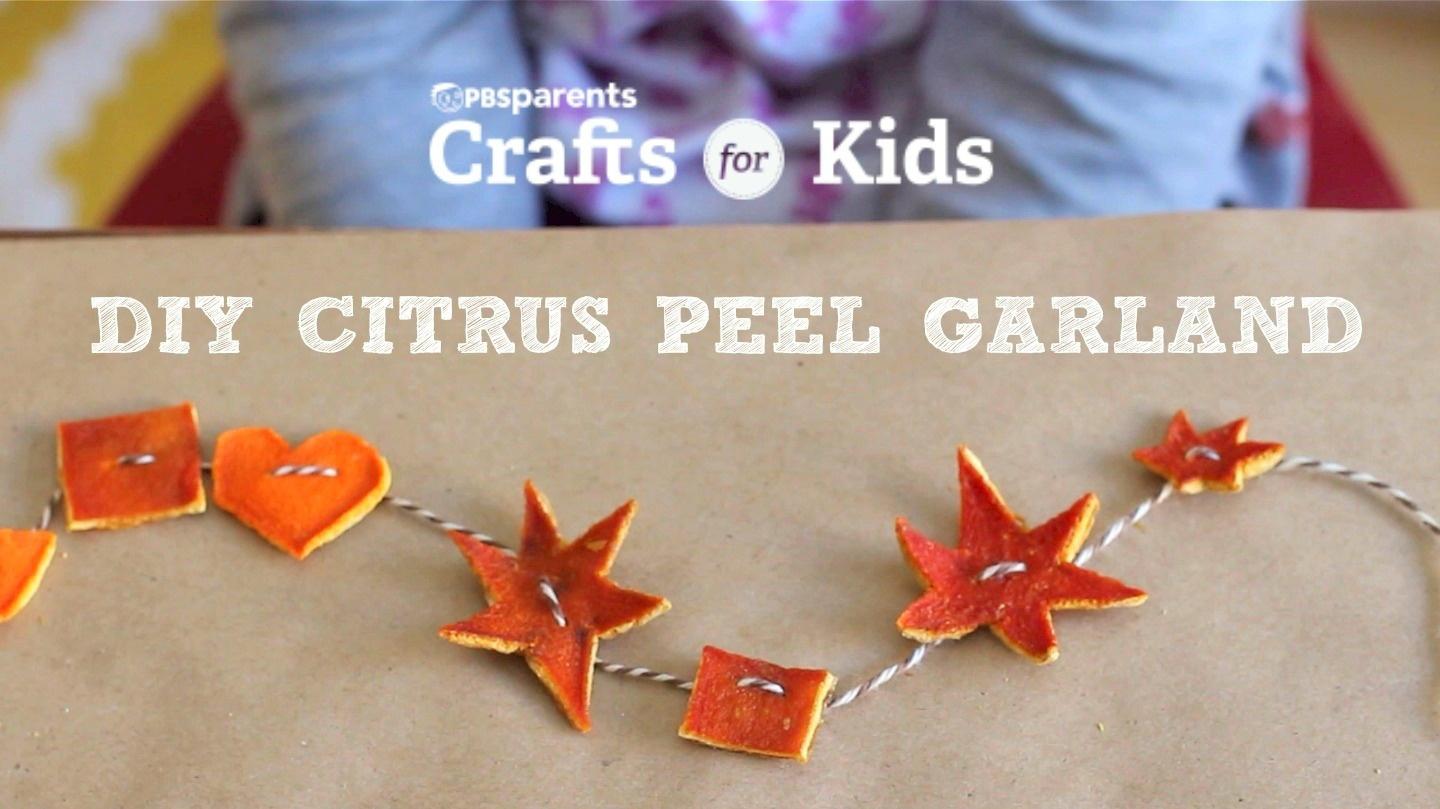The image is a landscape-oriented color photograph, showcasing a DIY citrus peel garland craft for kids. The bottom three-quarters of the picture features a light tan to brown table, where a rope of white and tan cord stretches from the left to the right side. Common shapes, including squares, hearts, stars, and rectangles, made of dried orange peel, are threaded onto the cord, arranged in a sequence of square, heart, starburst, rectangle, starburst, and small starburst. These shapes lie flat and are neatly displayed on the table's surface. Above the garland, in a slightly off-center, bold white stencil font, the text "DIY Citrus Peel Garland" is prominently visible. At the very top of the image, against a blue and multi-colored backdrop that includes hints of blue, white, purple, yellow, and red, is a partly visible child, identifiable by their gray long-sleeved garment seen from mid-elbows to mid-arms. In the center, a white text area features "PBS Parents" in smaller text and "Crafts for Kids" in larger text below it, with "for" displayed in dark text against an opaque white circle. The overall style of the image merges photographic realism with illustrative text to create an engaging and informative craft advertisement.